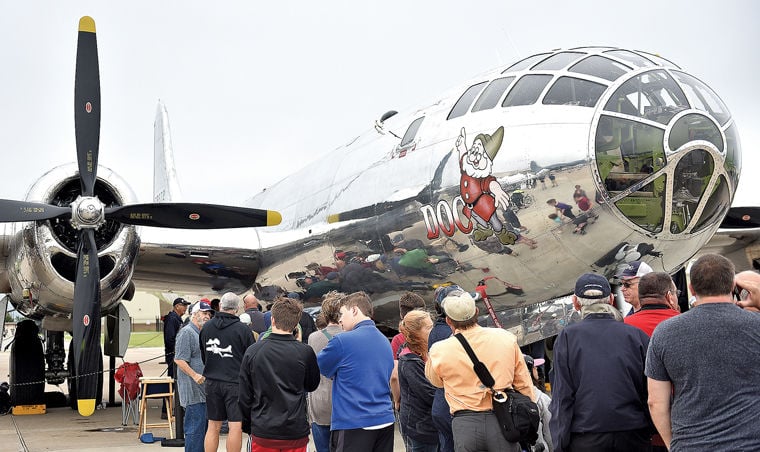The photograph depicts a shiny, chrome-plated airplane with a black propeller featuring yellow tips, positioned on the right engine. The aircraft's reflective surface mirrors the group of people standing on the ground below it. The fuselage showcases a vibrant design of Doc, a character from Snow White and the Seven Dwarfs, complete with his distinctive glasses, red suit with buttons, black belt, and a brown hat, pointing upwards. The word "Doc" is prominently displayed in white and red next to the character. Surrounding the plane are men and women, some possibly tourists or exhibit visitors, casually dressed in t-shirts, sweaters, and carrying backpacks. Their reflections are clearly visible on the lustrous surface of the plane. The background is a white sky, with various colors such as black, white, gray, red, yellow, blue, and orange accentuating the scene. The cockpit area features numerous windows, offering a glimpse inside.